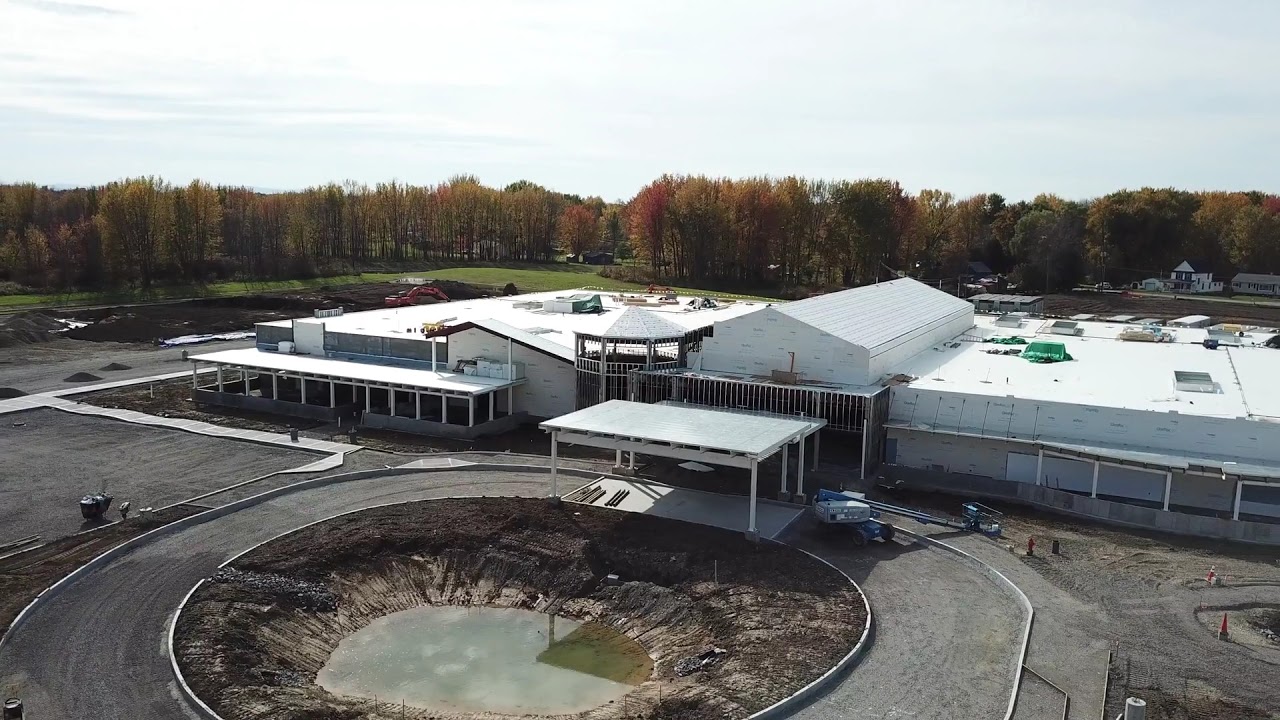This aerial view showcases a large, predominantly white building complex, suggesting a farm with several horse stables. At the entrance of the complex, a crane stands out, hinting at ongoing construction work. The entrance leads into a circular loop road, which surrounds a central median filled with brown dirt and a sizable pool of water, resembling a crater or a meteor impact site. The road circling this central area appears to be made of gray gravel. To the far right, construction cones can be seen, adding to the impression of an unfinished site. The building itself features a steel roof and a rooftop awning supported by pillars. Surrounding the complex, expansive green grass fields and a dense wooded area with multicolored foliage—reds, browns, and golds—indicate that it is likely autumn. Overhead, the sky is a mix of white and light blue, completing the serene landscape.